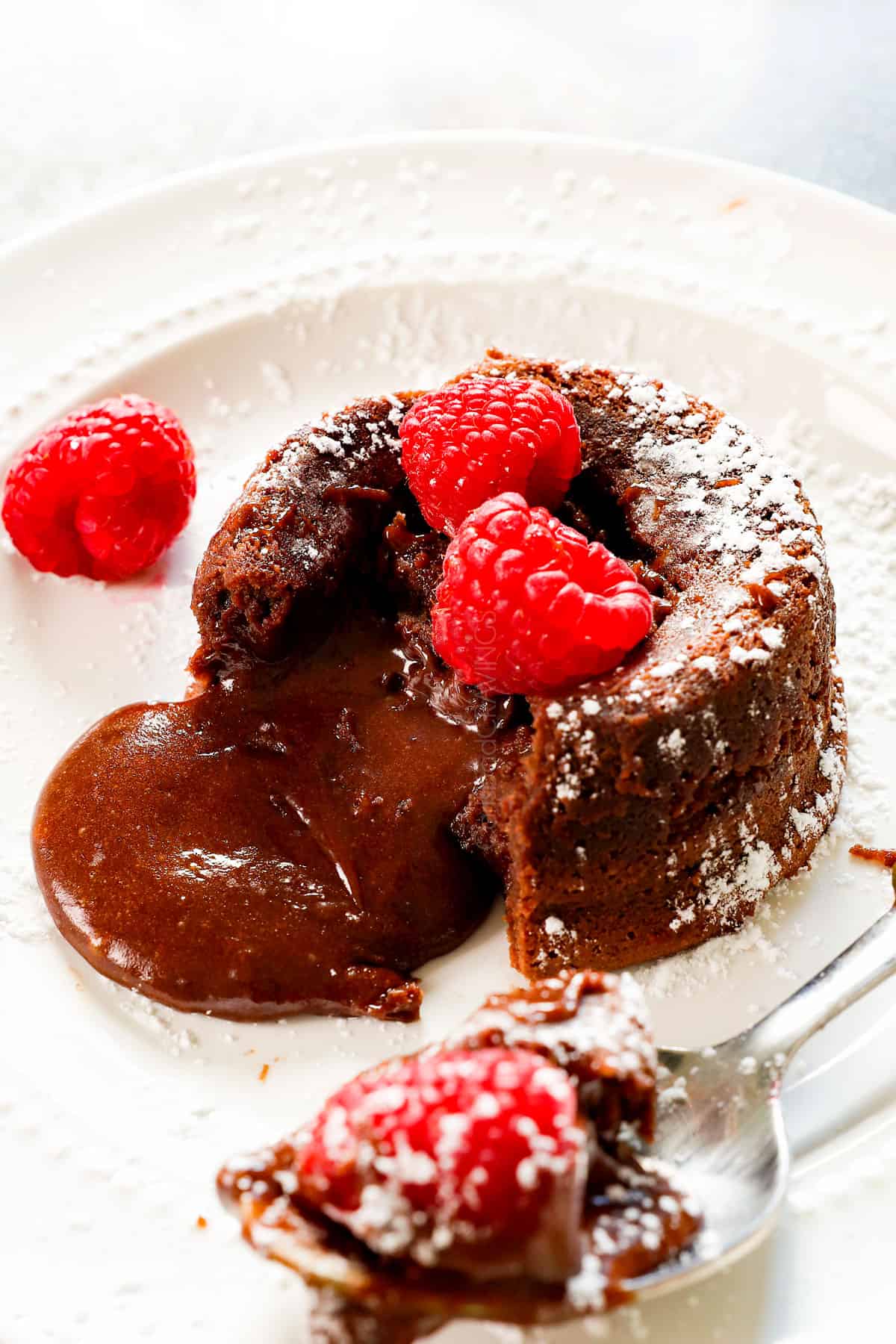A decadent molten chocolate lava cake sits elegantly on a white plate with an indented center and a dot pattern along the rim. The cake, dusted with powdered sugar, is split open, revealing rich chocolate oozing out to the left. Adorning the cake are three plump raspberries, two perched on top and one nestled beside it. A silver spoon in the foreground holds a luscious piece of the cake and a raspberry, poised against a bluish-grayish table. The presentation, enhanced by the powdered sugar scattered both on the cake and the plate, creates a visually enticing dessert tableau.